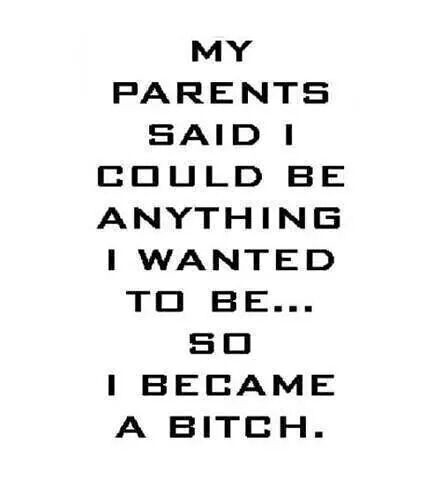The image features a plain white background that could belong to a sheet of paper, a t-shirt, or a white wall. In the center, black text is prominently displayed in an all-capitalized, squared-off font. The message reads, "My parents said I could be anything I wanted to be... So I became a bitch." The text uses an ellipsis to lead from the first sentence to the punchline. The simplicity of the design leaves the exact medium ambiguous, but the strong, clear font and stark contrast between the black text and white background make the message stand out distinctly.